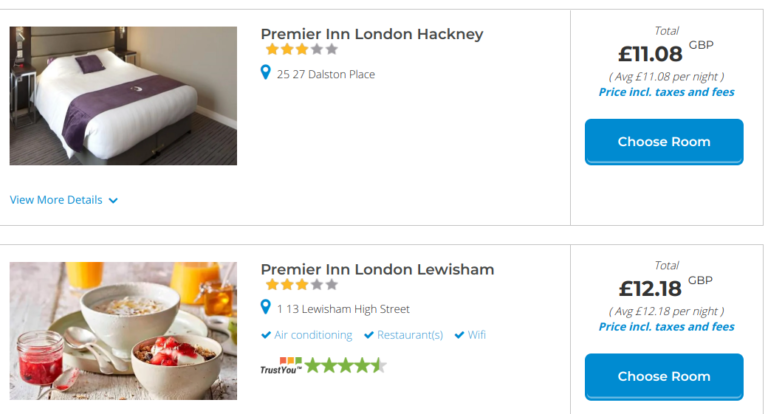The screenshot from an online application features two rows of listing previews, each showcasing an image and corresponding details for accommodations in London.

In the top row, positioned on the left side, there is an image of a neatly made bed situated in the corner of a room with light gray walls. The bed is adorned with white and dark brown striped bedding, complemented by a dark brown pillow. To the right of the image, the listing is labeled as "Premier in London Hackney." Adjacent to this label is the price, stated as £11.08 GBP. Beneath the price information, a blue rectangular button with the text "Choose Room" in white is clearly visible.

In the second row, there is an image showcasing a breakfast arrangement with food items presented in white bowls. Next to this image, the listing is identified as "Premier in London Lewisham," similar to the format seen in the top row.